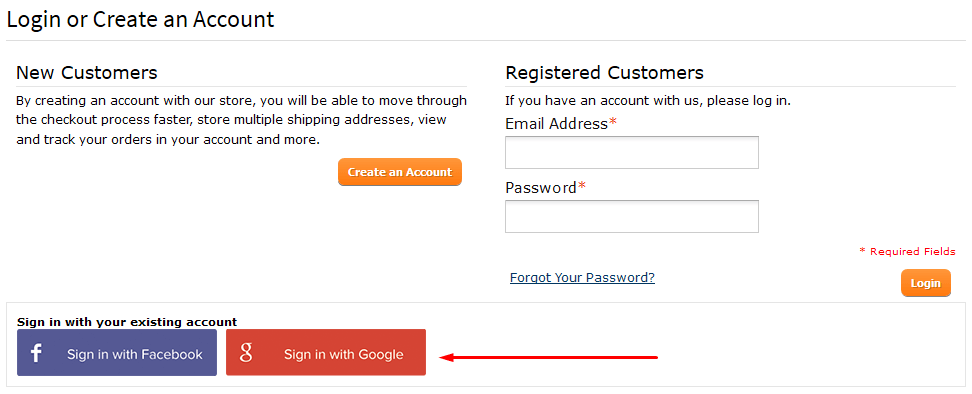This screenshot showcases a website login and account creation page, set against a clean, white background. At the top, there is a prominent heading that reads "Login or Create an Account." Below this, the section for new customers is introduced, outlining the benefits of account creation with the text: "By creating an account with our store, you will be able to move through the checkout process faster, store multiple shipping addresses, view and track your orders in your account, and more." 

An eye-catching orange button labeled "Create an Account" is situated beneath this informative text. To the right of the new customer section, the page prompts registered customers with "If you have an account with us, please log in." This section has input fields for "Email Address" and "Password," both marked with a red asterisk to indicate required fields. Between these input fields, there is a reminder option "Remember Me." Below the password field, a link allows users to "Forgot Your Password?" and adjacent to this link, there is a note explaining the asterisk denotes required fields.

Further down, an orange "Login" button invites users to sign in to their existing accounts. An alternative sign-in option encourages users with the text "Sign in with your existing account," highlighting social login options. Within a blue box is the Facebook logo accompanied by the text "Sign in with Facebook." Similarly, a red box featuring the Google key logo offers the option "Sign in with Google." A long red arrow directs attention specifically to the "Sign in with Google" button, emphasizing its availability as a login method.